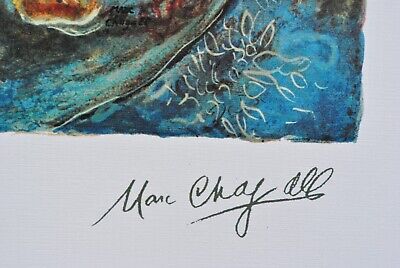The image captures the lower right corner of a partially visible piece of artwork by Marc Chagall. The dominant color in this section is a rich blue, with accents of white that resemble leaf-like sketches. Additionally, there are golden, feathery shapes positioned towards the bottom of the artwork. An elegant black cursive signature, reading "Marc Chagall," is prominently displayed in the corner, signifying the artist's autograph. The artwork is bordered by a white margin, which is notably thicker at the bottom, framing the fragment of the painting and emphasizing the signature. Hints of orange and a patina of blue and green hues add to the intricate details, making this snippet a beautiful and intriguing glimpse of Chagall's larger work.